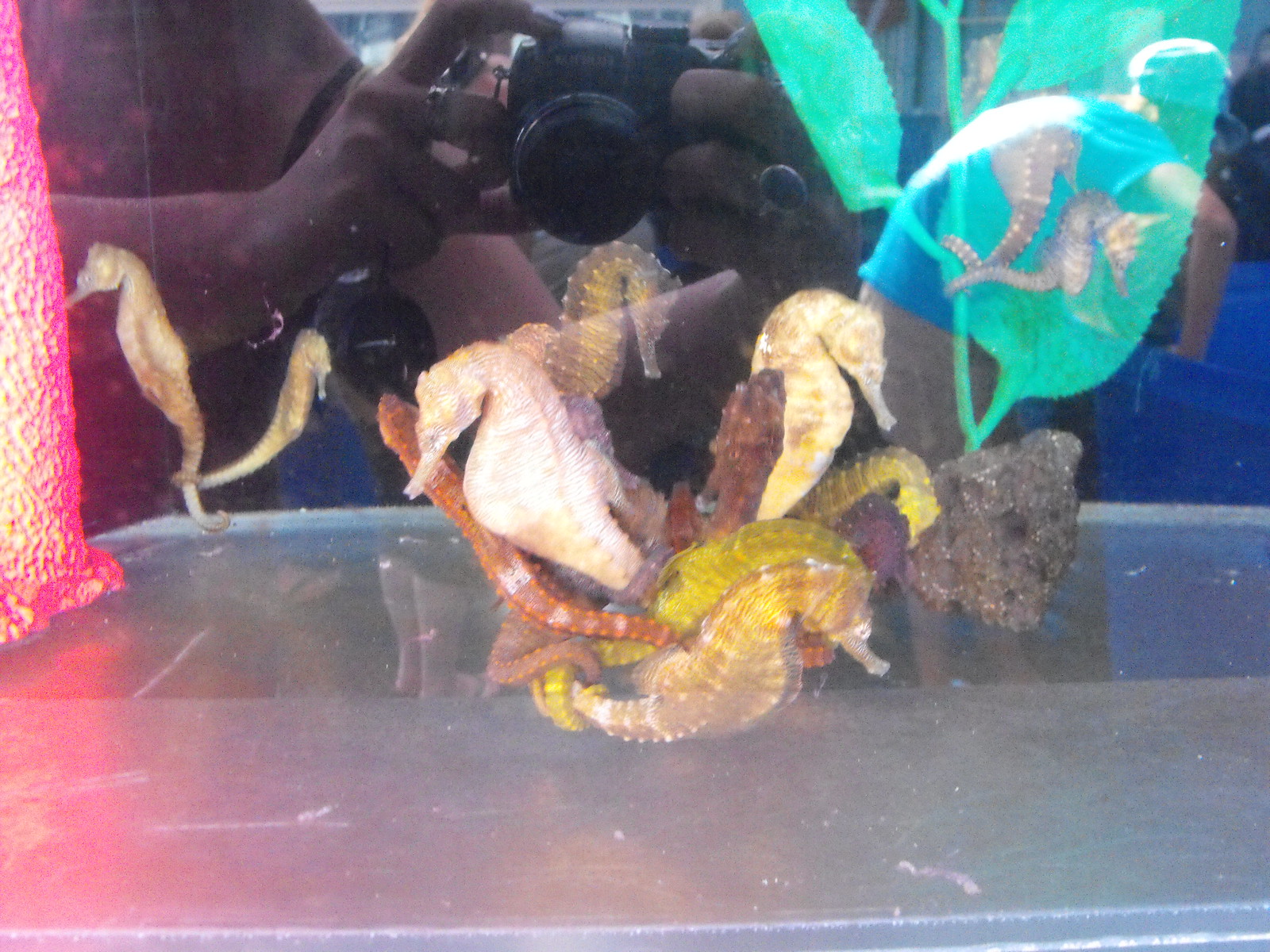The vivid scene captures a variety of seahorses floating gracefully in a large aquarium, each showcasing unique colors—including a white seahorse with a grayish back, a yellow patterned seahorse, and a green seahorse. In the foreground, two light brown seahorses are entwined, holding each other's tails next to a piece of lava rock. Nearby, two more light brown seahorses are wrapped around an underwater plant with broad, light green leaves. The gray rocks at the bottom add depth to the scene. Reflected in the aquarium glass, you can see the silhouette of the photographer holding a digital camera, focusing on capturing this marine tableau. Beyond the glass, a workman in a blue shirt, beige shorts, and a ball cap is busy with a blue tarp or a large plastic bin, adding an intriguing human element to the serene underwater display.